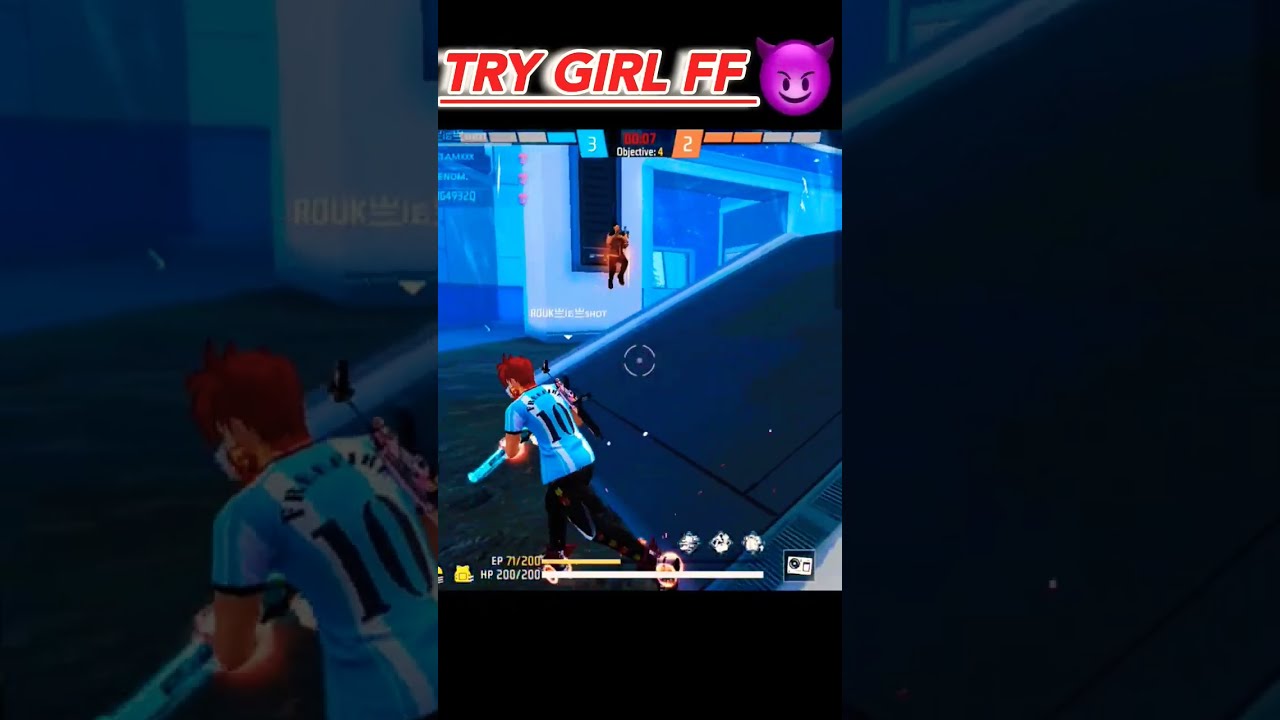The screenshot captures a dynamic scene from a mobile game. Prominently displayed at the top are the bold, red and white words "TRY GIRL FF," accompanied by a mischievous purple devil emoji with horns. Below this header, the screen shows a score of 3 to 2, indicating an ongoing match with just seven seconds remaining. Identified as a third-person shooter game, the environment features digital blue buildings and grassy terrain. The main character, clad in a blue soccer jersey and black pants, is depicted crouching behind a large wall. This character has a full health bar, reading "HP 200/200," and an experience points bar labeled "EP 71/200." In the backdrop, another character dressed in brown appears to be floating or hovering. The immersive graphics and detailed interface, laden with various colored bars and intricate stats, enrich the gaming experience further.